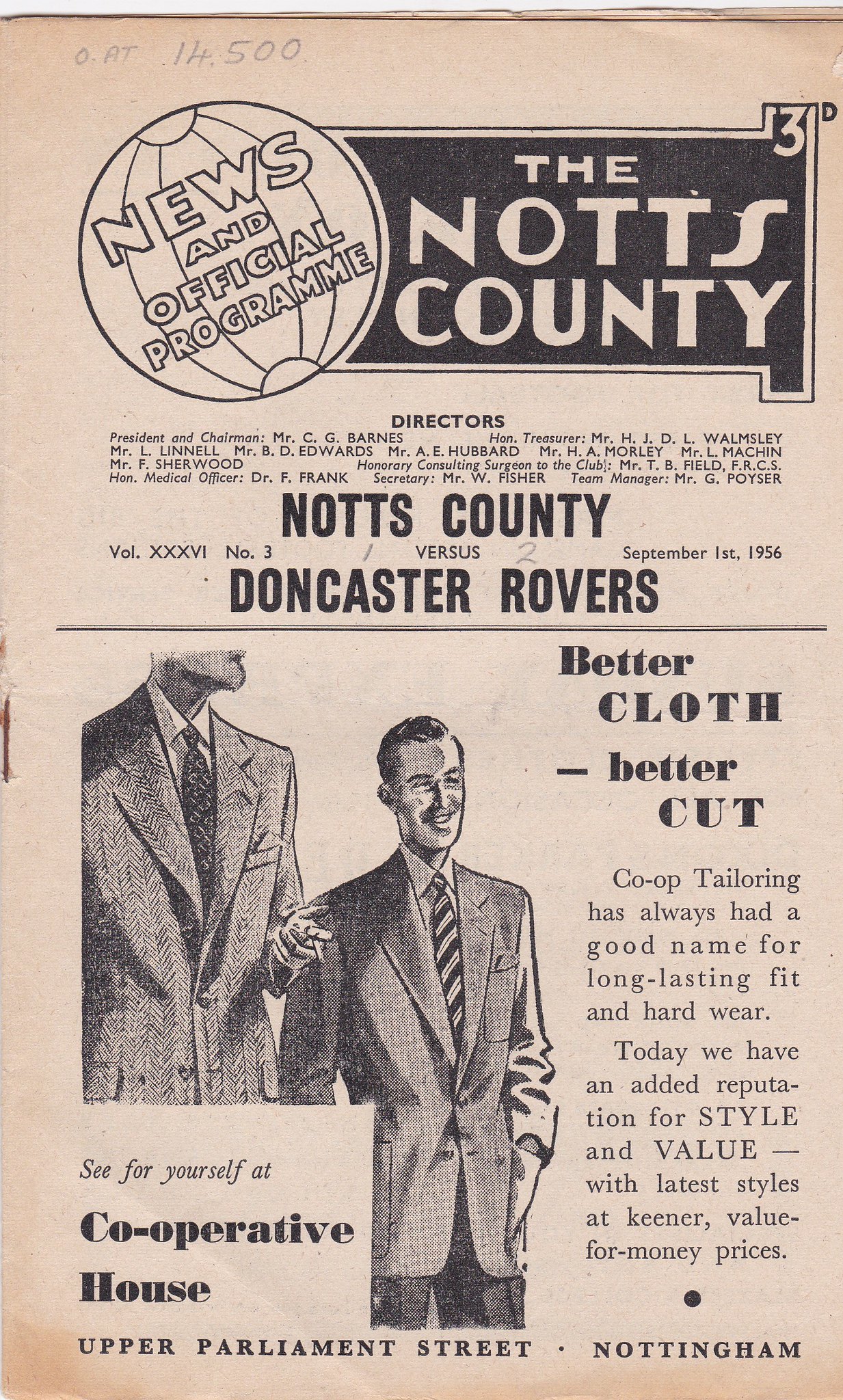The image portrays a vintage advertisement that appears to be from a publication dated September 1, 1956, quite possibly related to a football match between Knotts County and Doncaster Rovers. The primary background colour of the page is a peach tone, with a black banner at the top featuring the title "Knotts County News and Official Programme." Beneath this, the headline "Knotts County versus Doncaster Rovers" is prominently displayed in bold black text. To the left, there is an illustration resembling a beach ball.

A charcoal or pencil drawing of two men in suits occupies the lower part of the image. The men, with only one head visible, are advertising the suits themselves, complemented by the slogan, "Better Cloth, Better Cut." The accompanying text praises the Co-operative House on Upper Parliament Street, Nottingham, highlighting the co-op tailoring for its long-lasting fit, hardware, style, and value. The vintage ad, with its aged appearance in black and white with a brown pamphlet background, blends both the allure of sophisticated men's suits and the excitement of an upcoming football match.